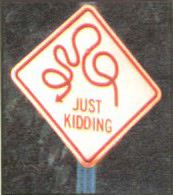The image showcases a road sign positioned on a gray metal pole, with a backdrop of indistinct trees and vegetation, lending a somewhat blurry and dark ambiance. The sign itself commands about 70% of the frame. It features a square shape aligned diagonally, presenting a diamond appearance. Dominated by a white background, the sign is encased in a red border close to its edge. A striking red squiggly line winds through the center, forming four loops and culminating in an arrow on the right. Beneath this playful design, the words "JUST KIDDING" are emblazoned in bold red letters. The overall scene hints at a humorous twist on typical road signs, suggesting curves ahead only to amusingly negate the warning.